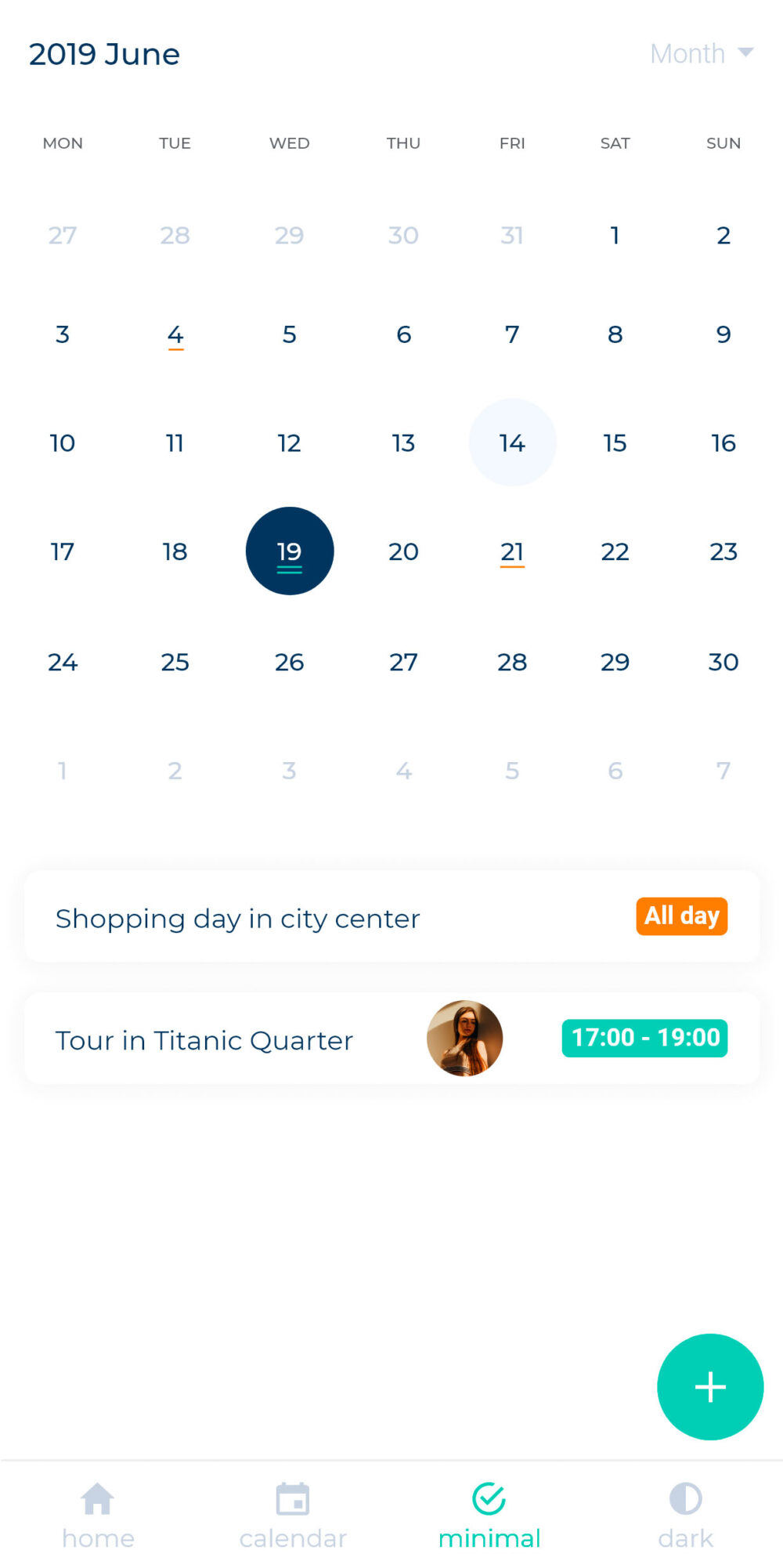This image depicts a personalized digital calendar for June 2019. The days of the week—Monday, Tuesday, Wednesday, Thursday, Friday, Saturday, and Sunday—are abbreviated and arranged horizontally across the top. The month of June is selected via a dropdown menu, revealing that the first day of June fell on a Saturday and the last day, the 30th, on a Sunday. A preview for the following month includes the first four days of July, with a special note that the 1st is marked as "Shopping Day in City Center" in orange.

A notable entry on the calendar is for the 19th of June, which is circled in blue and includes a time slot between 17:00 and 19:00 for a "Tour in Titanic Quarter." An image of a woman accompanies this entry. The calendar features customizable settings, allowing users to choose between themes such as "Home," "Minimal," and "Dark" to tailor the appearance of their personal scheduler. This organized and detailed calendar enables the user to plan and refer to their schedules throughout the month effectively.